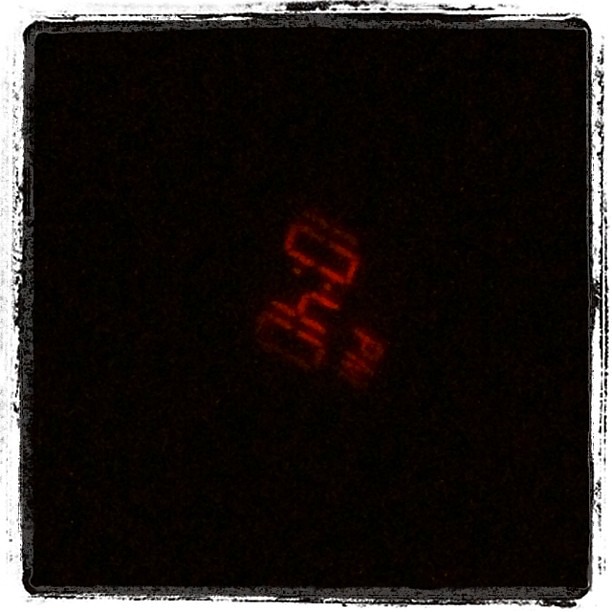A haunting photograph captures the faint glow of a digital clock readout, set against a pitch-black background. The image, tinged with a distressed and faded outline, evokes a sense of eerie emptiness. Positioned slightly askew and off-center, the clock displays the time "10:40 p.m." in a luminous, yet blurred, green text. The small, glowing digits seem to float in the vast darkness, accentuating the desolate and obscure atmosphere of the photograph.